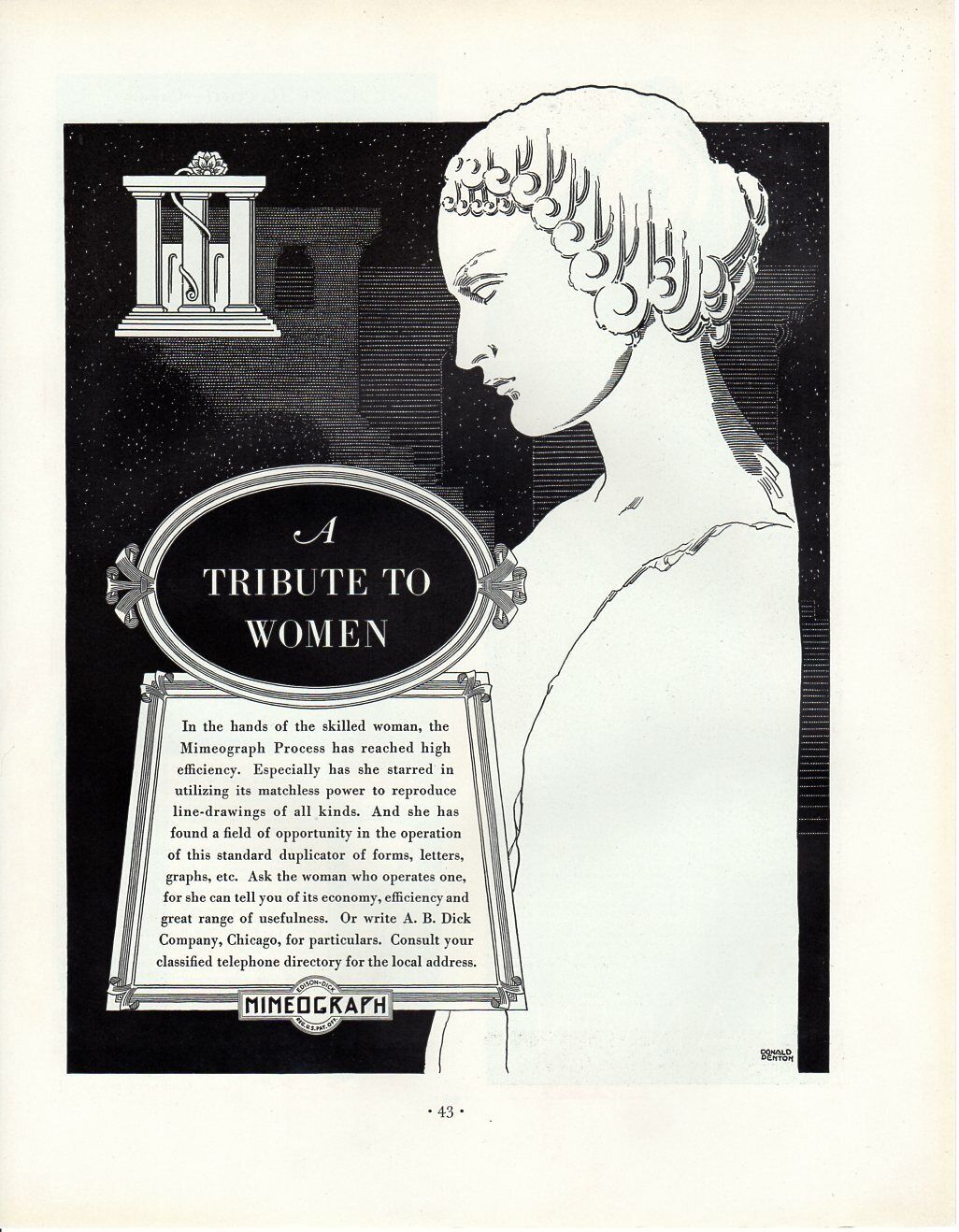The image is a black and white page from an old, discolored magazine or book. The central illustration features a classical scene with a colonnade consisting of three pillars with small stairs leading up to them. The central pillar has intricate details, including a vine or possibly a cat's tail with a puffy mane wrapped around it. To the right, a statue of a woman with short, curled hair stands sideways, looking to the left. The statue is primarily a plain white color, with detailed curls on its head.

The background of the page is black and features white etchings of classical architecture, including what appears to be a coliseum adorned with flowers and ribbon. At the center of the page, there is a black oval with a white text inscription that reads "A Tribute to Woman," with the "A" in cursive and the rest in capital letters. Below this oval, there is a square box framed in a dark black border, containing a paragraph of text. The text begins with "In the hands of the skilled woman, the mimeograph process has reached high efficiency" and further mentions the woman's matchless power to reproduce line drawings of all kinds. At the bottom of the square, the word "mimeograph" is highlighted in a small circle. Additionally, there is some small, unreadable text in the bottom right corner of the image.